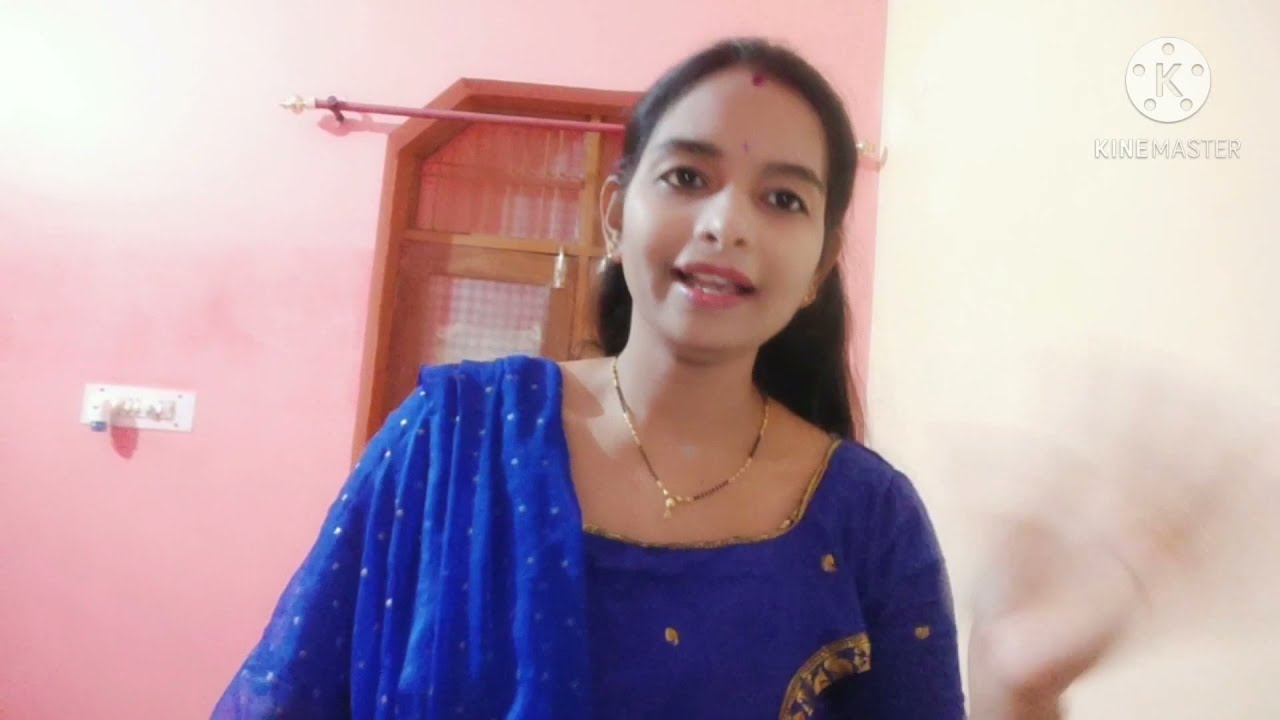The image depicts a smiling woman, likely Indian, with long brown hair, dark eyes, and dark eyebrows, wearing pink lipstick. She has a noticeable red bindi on her forehead and is accessorized with stud earrings, and a gold chain necklace with a small pendant. She is dressed in a bright blue top or dress adorned with gold trimming, and she has a blue throw around her shoulders. Her hand is raised in a waving motion, appearing slightly blurry. The background features a pink wall with white light switches and possibly a shelf, while a wooden door or window with a curtain rod (but no curtain) is visible behind her. In the upper right corner, there's a circular logo with a 'K' in the center and the word "KINDMASTER" written below it in white letters.